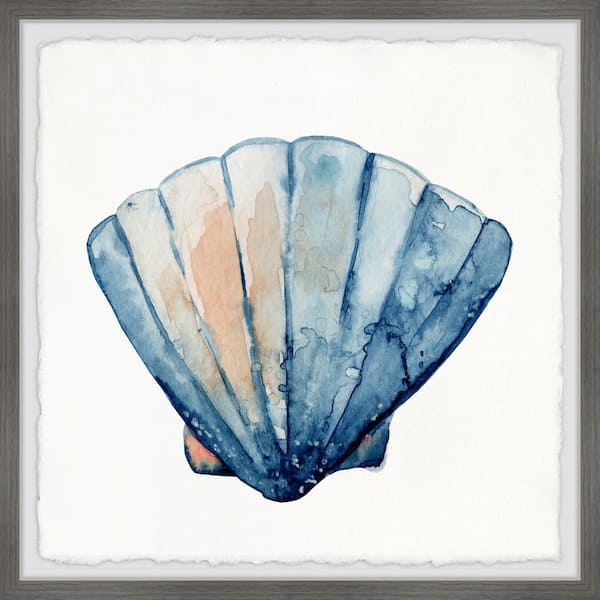This artwork features a watercolor painting of a blue scallop shell, centrally positioned on a bright white, slightly jagged-edged canvas. The shell, painted in varying shades of blue, transitions from dark blue at its base to lighter blue towards the edges. It includes additional splashes of white and orange-brown, lending a worn, weathered appearance. Surrounding the canvas is an off-white mat, and the entire piece is encased in a dark gray, wooden frame approximately half an inch thick. The background is simple and devoid of other elements, highlighting the shell's vibrant, high-contrast colors. The piece remains unsigned, leaving the artist anonymous.